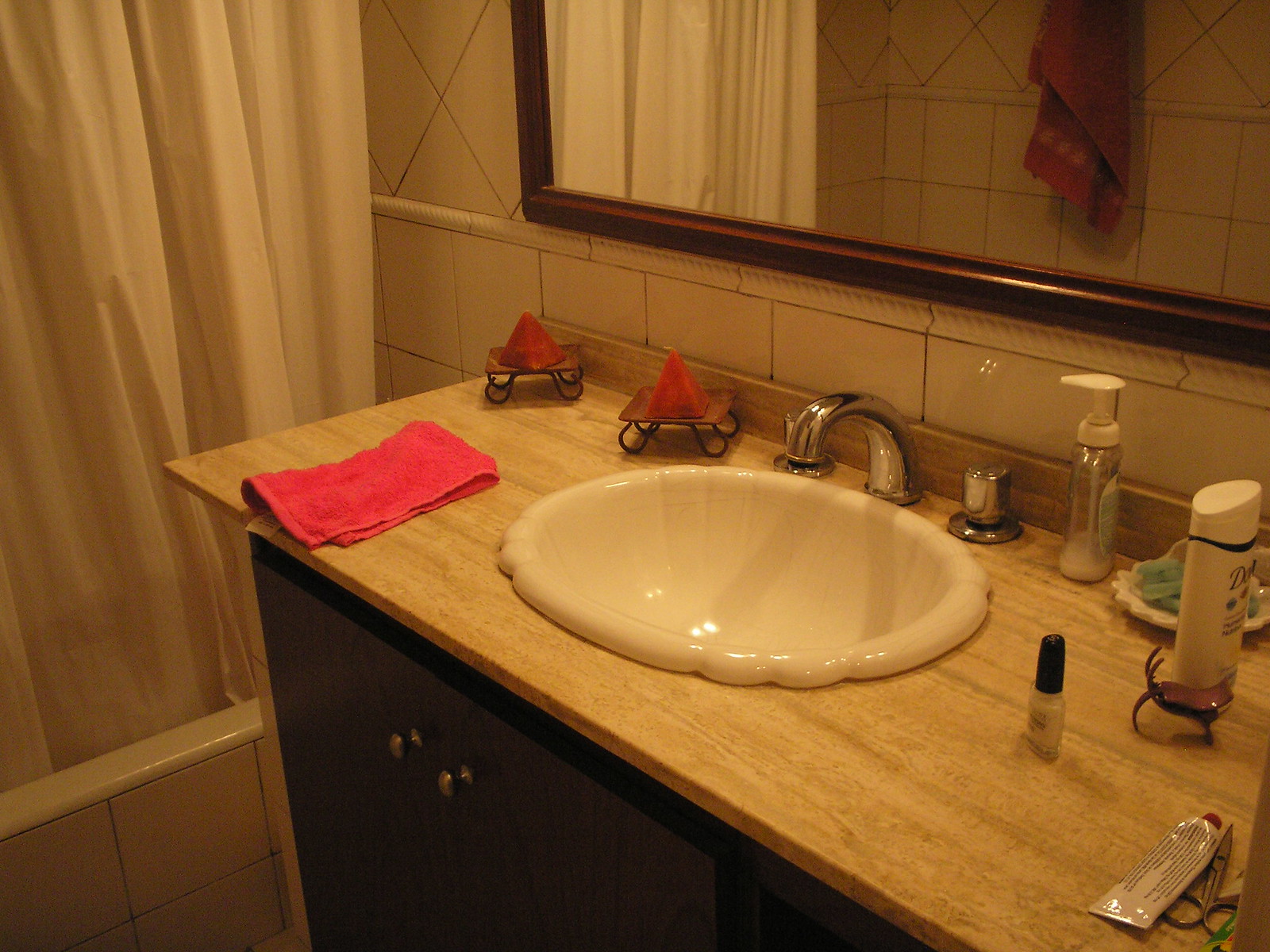A quaint and outdated bathroom vanity hosts a shell-shaped sink bowl, surrounded by a variety of personal items. Above, a large mirror reflects the room, while holders around the sink keep necessities organized. Scattered across the vanity are a nail polish, a soap holder, deodorant, lotions, and a pair of scissors, giving a glimpse into daily routines.